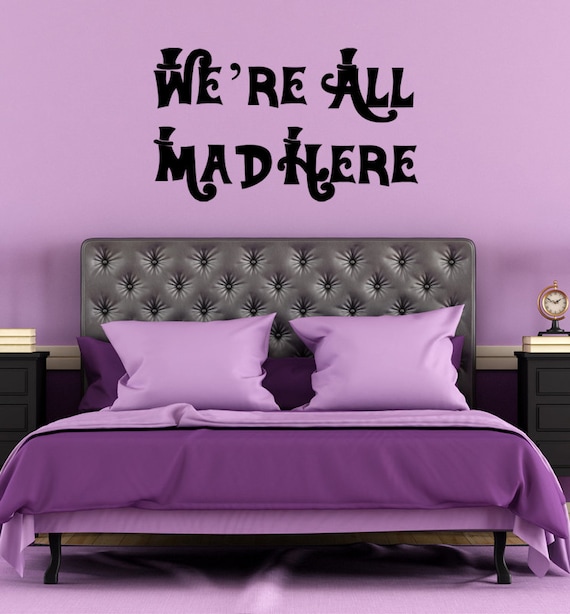The photograph showcases a striking purple-themed bedroom centered around a black upholstered bed with a shiny, quilted headboard, possibly made of leather or vinyl. The bed is dressed in various shades of purple, including a deep purple duvet, lilac sheets, lighter purple pillows, and dark purple shams, all resting on a purple rug that matches the bedding. Above the bed, the wall is decorated with black text that reads "we're all mad here," with a whimsical touch of small black top hats adorning the capital letters W, A, M, and H, reminiscent of the Mad Hatter from Alice in Wonderland. Flanking the bed are two dark gray (or ebony) side tables; the right table holds two books and a small round pedestal clock showing the time as ten after ten, while the left table supports a stack of three books. The room’s wooden flooring is partially visible beneath the bed, adding to the visual detail of this distinctly themed space.